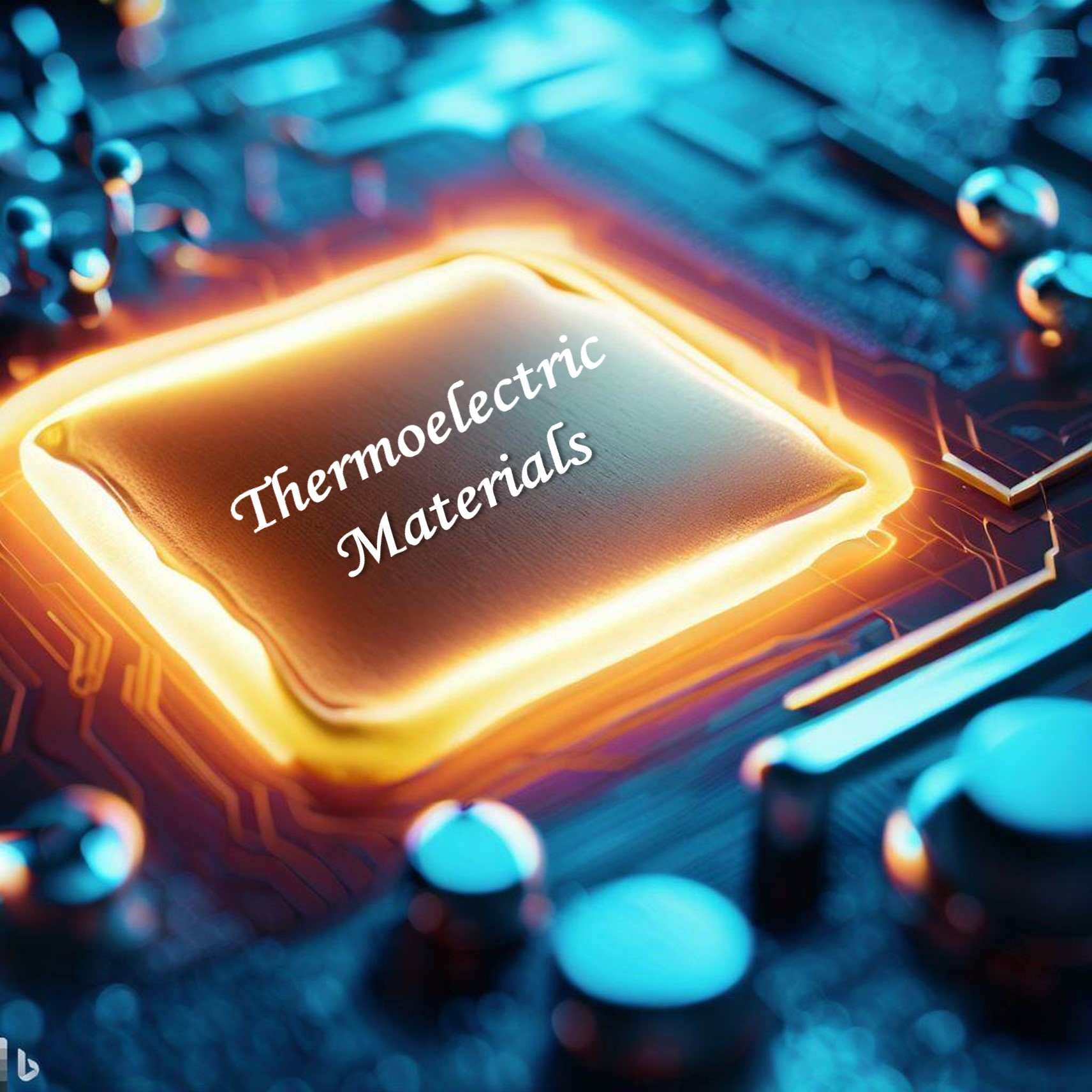The image features a meticulously edited square photograph showcasing a central glowing element, likely enhanced using software such as Photoshop. The background is a rich blend of blue, aqua, and black hues, depicting a blurred array of electronic components. These components include what seem to be computer chips, capacitors, rods, and other elements in shades of silver and blue. Positioned prominently in the center is a square with an intense orangish-yellow glow, resembling a CPU or a specialized thermoelectric device.

This central glowing square features a black section with white italicized text in two lines: the first line reads "thermoelectric" and the second "materials." Surrounding this are intricate details of the circuit board in striking blue, with the CPU-like component emitting a "white-hot" radiance along its edges. Additional features include silver-toned button-like elements with a slight blue tint dispersed around the glowing square. The overall composition suggests a high-tech theme, possibly serving as an advertisement, promotional material, or even a book cover highlighting thermoelectric materials and technology.